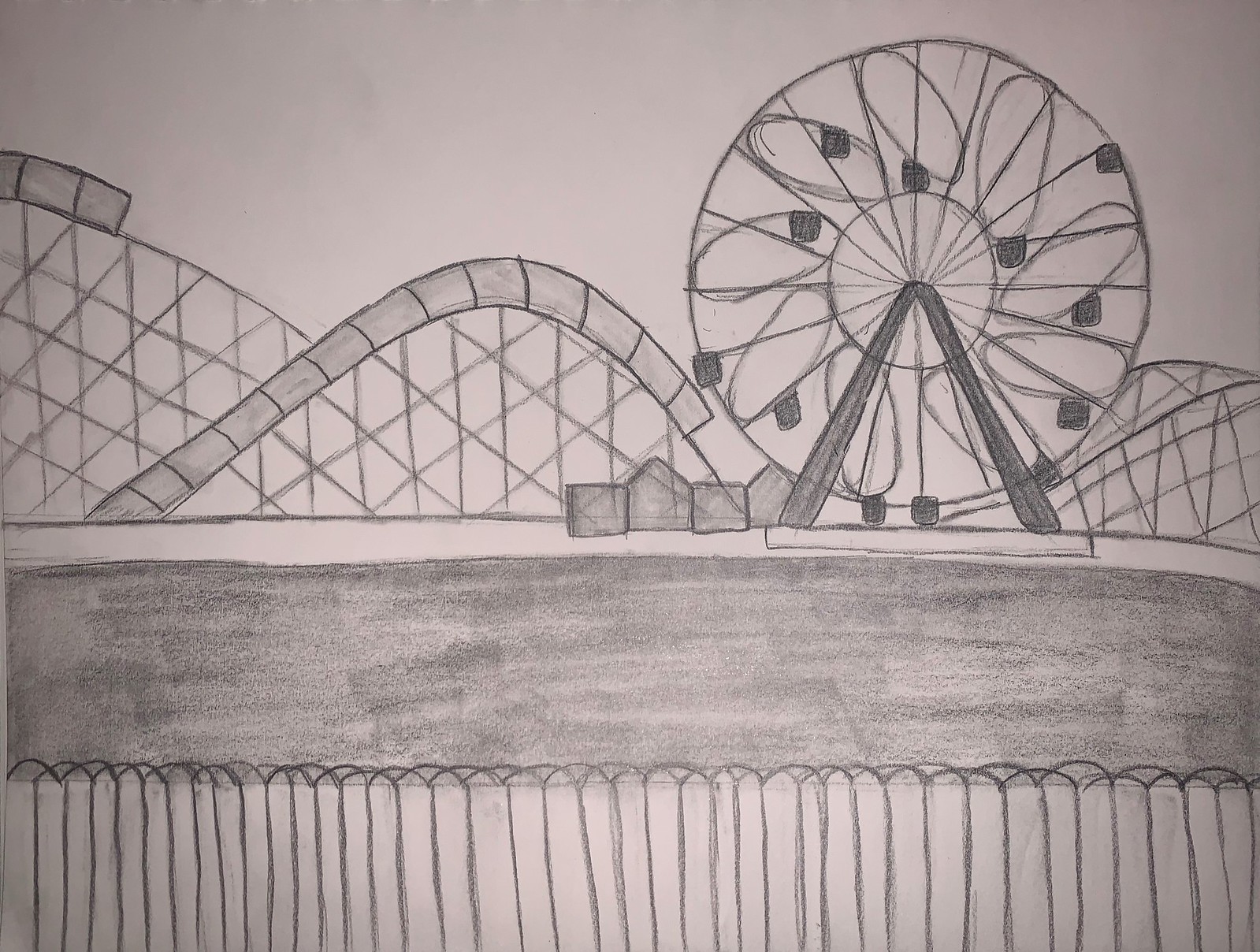This detailed pencil sketch of an amusement park features prominent attractions and thoughtful shading. In the forefront, there's a wooden-paneled fence providing a barrier to the scene. Just beyond the fence, shaded areas depict what could be pavement or grass. Dominating the top right of the drawing is a Ferris wheel, characterized by intricate details such as spokes, an inner circle, and rectangular or circular carriages. This Ferris wheel is supported by a triangular framework. Behind it, a sprawling roller coaster weaves from the left to right, boasting two prominent hills on the left and one on the right. A building sits in front of the roller coaster, adding depth to the sketch. Textural hatching beneath the roller coaster suggests a classic wooden structure. The entire scene is set against the contrast of white paper, with the use of grey and black to add dimension and realism. The sketch style captures the essence of an amusement park from a distant perspective.